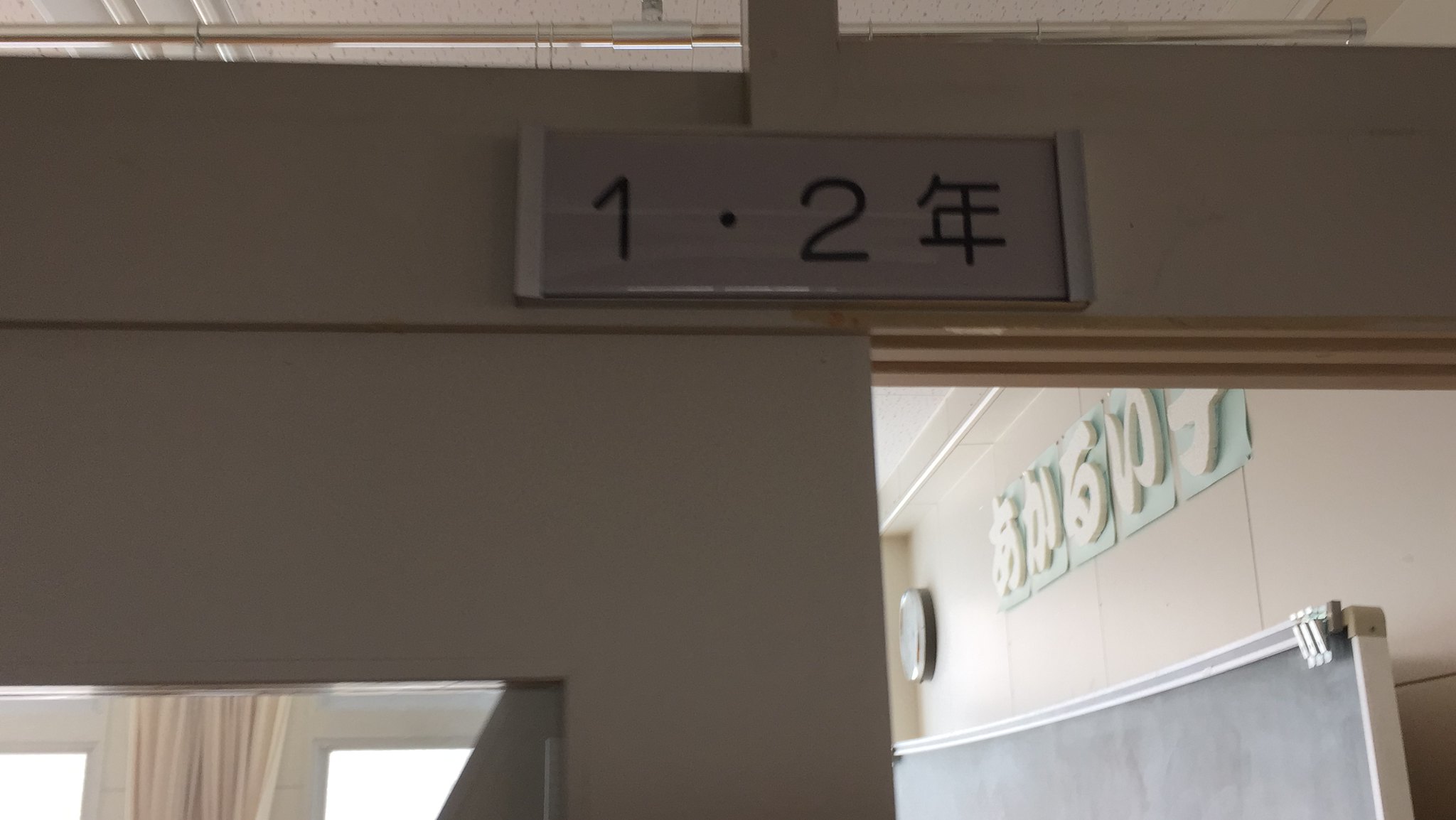This color photograph captures an upward-angled view starting from the lower left-hand corner, revealing a partial door and the number "12" followed by a character, possibly in Chinese or Japanese. A glimpse inside the room, seen in the lower right-hand corner, shows an old-fashioned gray chalkboard situated against a beige wall. Above the chalkboard, four unreadable letters are positioned at the wall's top. A wall clock's side profile is barely visible at the far edge of the image.